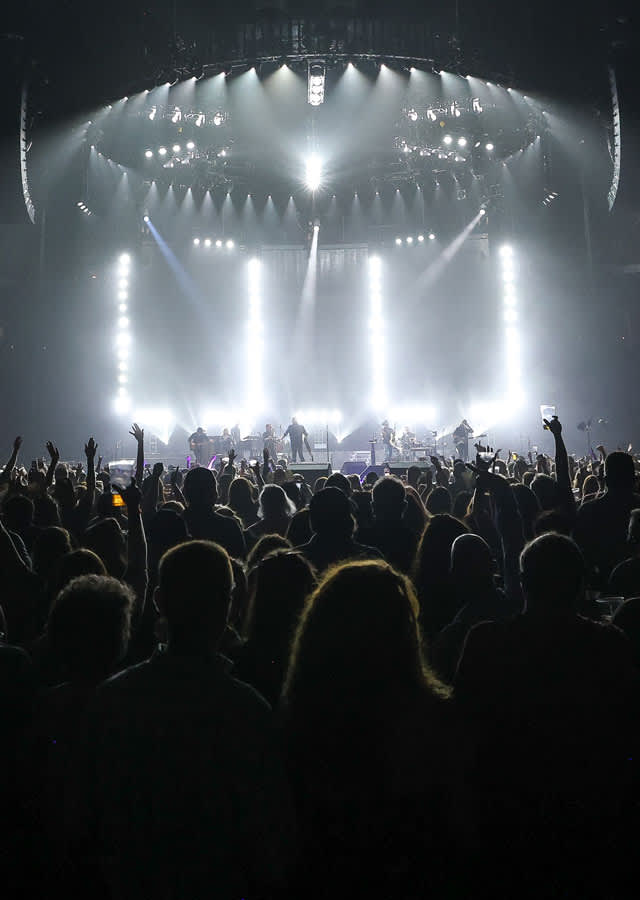The image captures an electrifying concert scene from a vertical perspective about 10 to 15 rows back in the audience. The darkness of the photograph is punctuated by vibrant spotlights and streams of light, with four columns of light dramatically illuminating the back of the stage and multiple diagonal spotlights enhancing the performance. The stage is lively with at least seven performers, including someone with a guitar and a visible drum kit. The crowd is immersed in the moment, their raised hands and drinks silhouetted against the glow of the stage lights. Directly in front, a woman with long hair and a man with very short hair are noticeable among the sea of enthusiastic concert-goers, many of whom are capturing the experience with their cameras. The atmosphere is one of sheer excitement and joy shared by everyone in attendance.